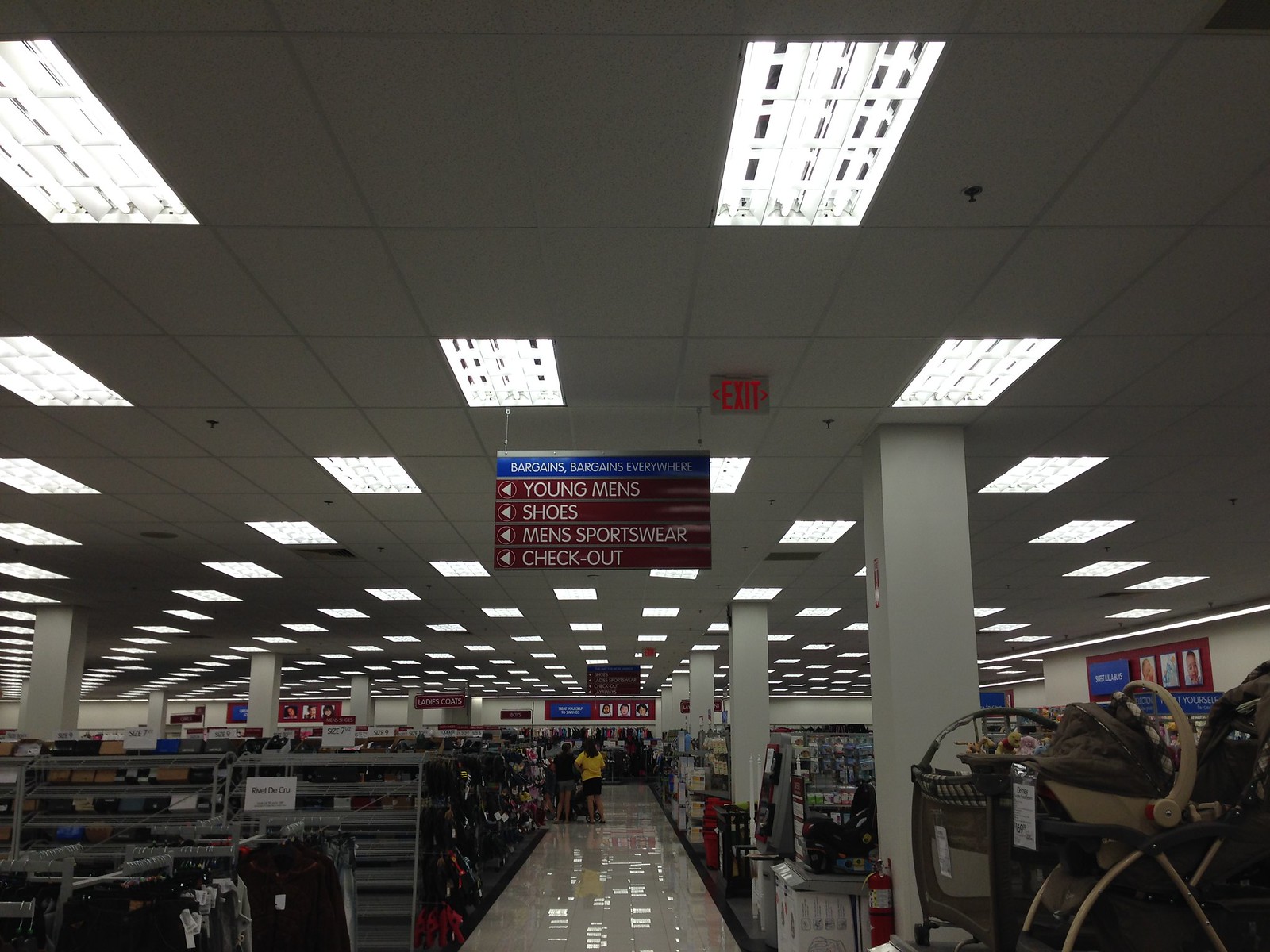The image depicts a well-lit retail store interior with various fixtures and signs. The ceiling is adorned with different types of modern lighting fixtures, and several square-shaped panels add an architectural interest. Hanging down from the ceiling are signs enclosed in red rectangles, each inscribed with white text and featuring left-pointing arrows, clearly directing shoppers to sections such as 'Young Men’s Shoes' and 'Men’s Sportswear'. The store floor is covered in reflective linoleum, enhancing the brightness of the space. 

In the foreground, substantial support pillars are visible, which both demarcate sections and support overhead shelving. These shelves are stocked with a variety of items, including baby strollers to the right, and an assortment of fabric materials. The visual layout and organization of products make navigation easy for customers, guiding them through different departments efficiently.